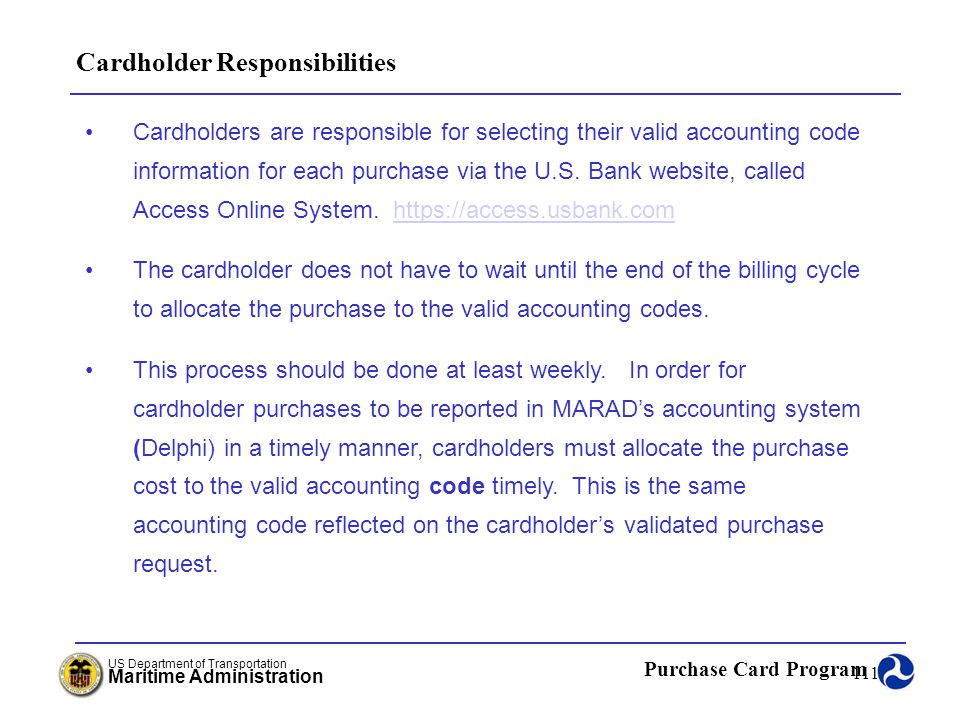The image displays a detailed PowerPoint slide or webpage content titled "Cardholder Responsibilities" in black text at the top, with an underline of solid blue. Below, in medium blue font, are three detailed bullet points. The first bullet point indicates that "Cardholders are responsible for selecting their valid account and code information for each purchase via the U.S. Bank website called Access Online System," followed by the specific website address. The second bullet explains that "The cardholder does not have to wait until the end of the billing cycle to allocate the purchase to the valid accounting codes." The third bullet point emphasizes, "This process should be done at least weekly in order for cardholder purchases to be reported in MARAD's accounting system (Delphi) in a timely manner. Cardholders must allocate the purchase costs to the valid accounting code timely. This is the same accounting code reflected in the cardholder's validated purchase request." Another solid blue line divides the content, below which on the lower left is the "U.S. Department of Transportation, Maritime Administration" logo, and on the lower right, it reads "Purchase Card Program" with a related logo featuring a black icon and a white swirl. The background of the entire image is white, ensuring the text is clear and readable.